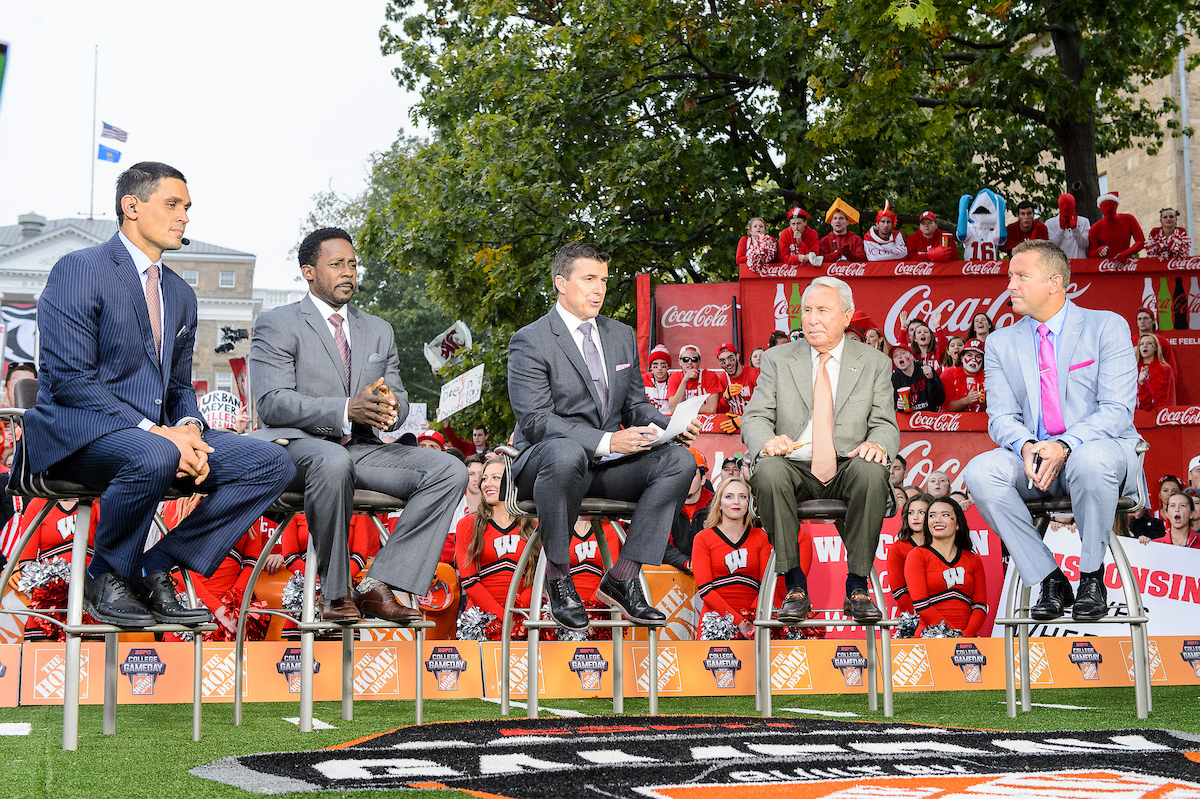The image depicts five male sports announcers presenting live from a college football show, typically aired on Saturday mornings. They are seated in high, bar stool-like chairs arranged in a semi-circle on a grassy surface, which features a painted logo and a sponsor's advertisement—likely by Home Depot—both on the ground and on a banner behind them. The announcers are all dressed in suits of varying colors including light blue, brown, gray, and navy blue, complete with ties and dress shoes. Behind them, a sizable crowd has gathered, and among them are Wisconsin cheerleaders in red sweaters with white "W" letters trimmed in black and red skirts, holding silvery pom-poms. The spectators, many of whom are wearing red jerseys with black collars, suggest a strong team presence. Additionally, visible in the background is a giant tree towering over the horizon, various red Coca-Cola signs with white lettering, signs, hats, and a distant building on the top left.